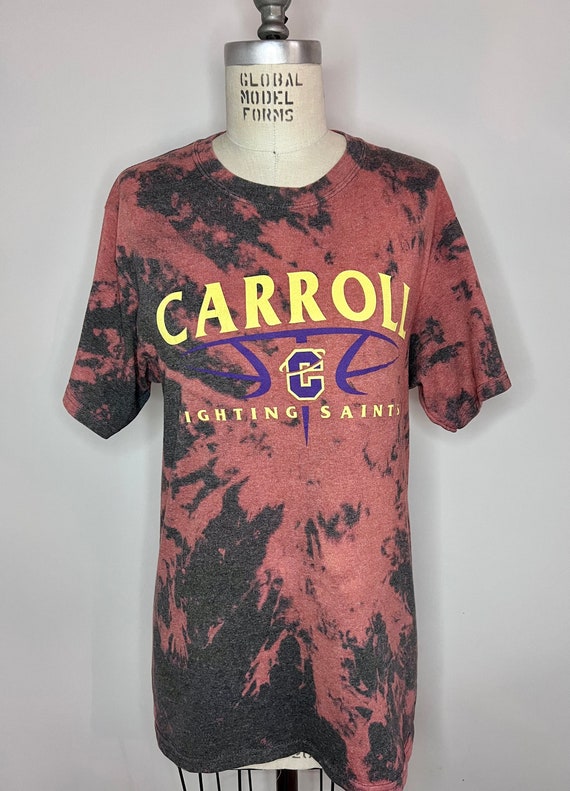The image features a t-shirt displayed on a mannequin torso, which is labeled "Global Model Forms" at the neck area in black stencil text. The mannequin has a silver cap where its head would be. The t-shirt itself is predominantly red and black with short sleeves. The chest area of the t-shirt prominently displays the name "Carol" in bold, yellow capital letters. Below this, there is a purple graphic with a large, capital letter "C" outlined in yellow in the center. The text "Lightning Saints" appears beneath the graphic, though it is partially cut off. The mannequin has a black bottom and top setting.